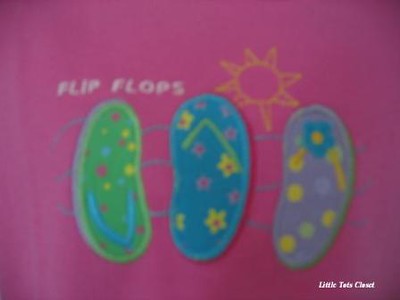This image depicts a detailed, colorful drawing that appears to be a t-shirt logo. Set against a blurred, hot pink fuchsia background, the design features three flip-flops with distinct decorations. The left flip-flop is green with multicolored polka dots and a blue thong. The middle flip-flop is blue with both yellow and pink flowers and has a green thong. The right flip-flop is purple with yellow polka dots, a yellow thong, and a blue flower between the toes. All three flip-flops are positioned atop three wavy lines. In the upper right corner, a bright yellow sun shines, while to the left of the sun, the word "flip-flops" is written in white text. Additionally, at the bottom right-hand corner, the phrase "Little Tets Closet" is inscribed, contributing to the playful and vibrant feel of the image.